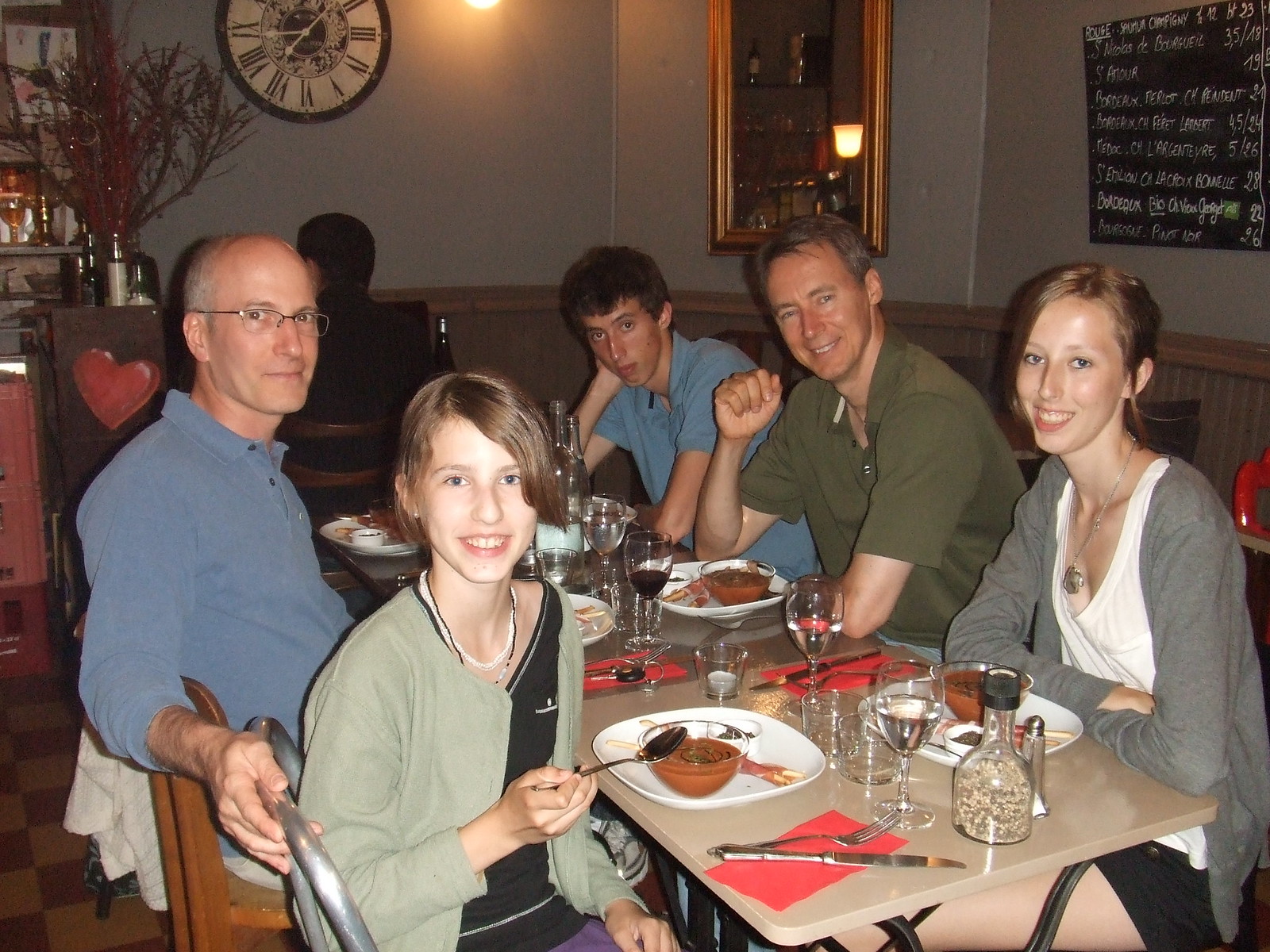In this detailed image, we see a family of five gathered in a restaurant, posed and smiling at the camera. The setting is clearly indoors, featuring a tiled floor and a rectangular dinner table at the center, adorned with plates, cups, glass goblets with water, silverware, and pink napkins. Each family member is distinctively described:

- On one side of the table, a young girl, likely a teenager with brown hair, is smiling warmly. She is wearing a green jacket over a black shirt and a necklace with white and black beads. In front of her is a bowl of pudding with a spoon resting on it, and a white plate beneath the bowl.
- Next to her, on her left, sits an older man with short gray hair, glasses, and a blue polo shirt. He appears relaxed, with his arm resting on her chair, and is also smiling at the camera.
- Across the table, on the right-hand side, a slender woman with a white tank top under a gray sweater is smiling gently. Her hands are crossed on the table, and she has not yet touched her bowl of pudding.
- To her left, another man, also with gray hair, wears a green polo shirt. He is smiling as well and has a glass goblet in front of him, possibly containing wine.
- At the edge of the table, to the left of this man, is a young boy, also a teenager, looking slightly bored with his face resting on his hand. He is dressed in a blue polo shirt.

The restaurant's interior includes gray-painted walls, a potted tree to the left, and a wooden chair adorned with a red heart. There's a clock with Roman numerals in the upper left corner, and a mirror at the center of the image. The table and seating arrangement are directly in the image's center, enhancing the family-focused composition. A chalkboard menu with writing is visible on the right-hand side, above the slender woman, adding to the cozy, casual dining atmosphere the image portrays.